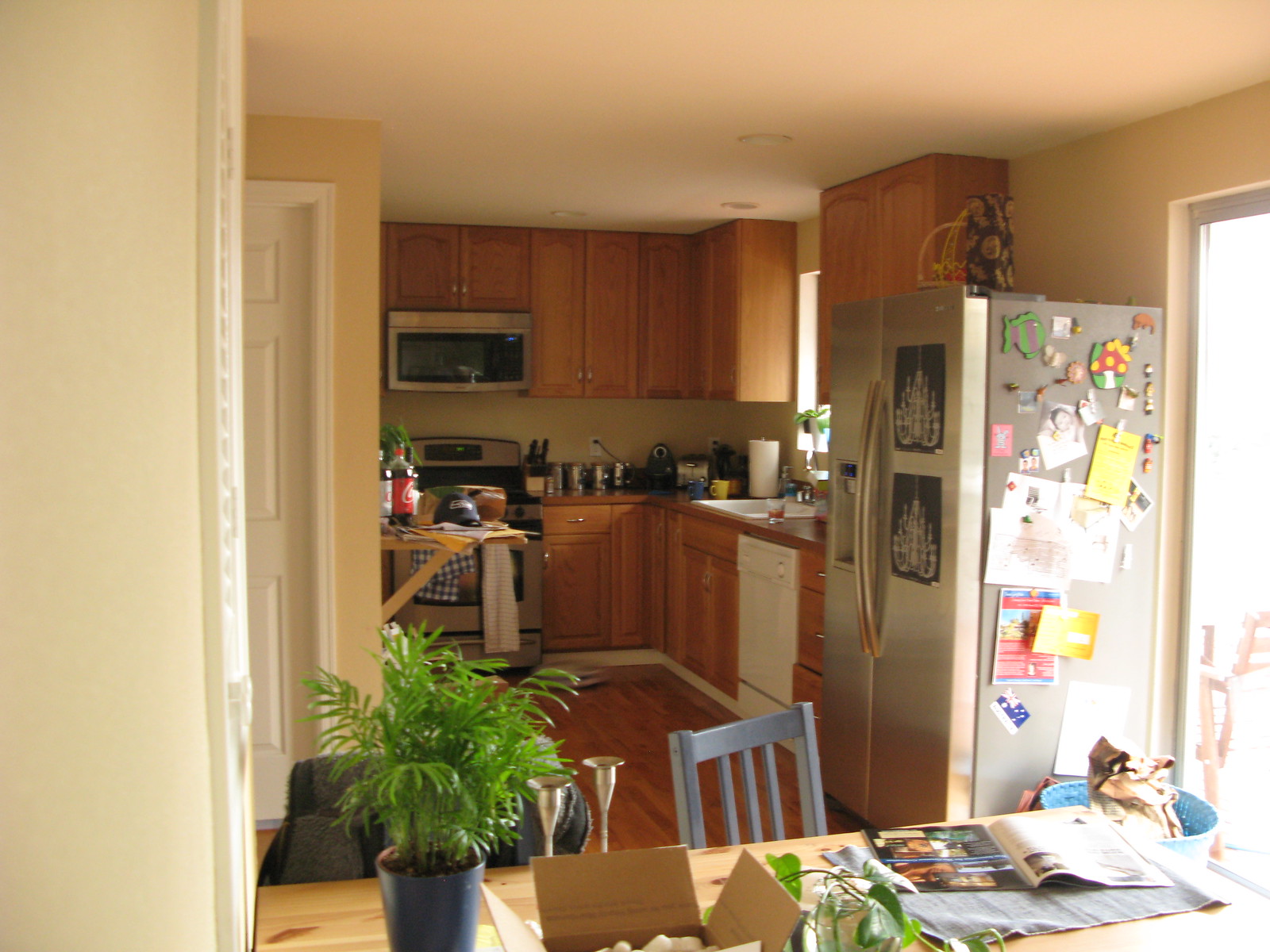In this modern kitchen, a cozy and somewhat cluttered dining scene unfolds. In the foreground, a wooden dining table is surrounded by blue wooden chairs. The table surface is scattered with various items, including scattered papers and an open magazine, giving a sense of casual everyday life. Beside these, a blue basket sits—its contents obscured—while a potted plant adds a touch of greenery. An open box on the table reveals packaging foam but conceals its contents. Dominating the background, a sleek, stainless steel refrigerator stands out, covered in a collection of magnets, notes, and pictures of animals, adding a personal touch to the modern aesthetic. Adjacent appliances, including a high-end microwave and a stove/oven combination, hint at the kitchen's functionality. A small pop-out tray, seemingly emerging from an unseen location, holds two-liter bottles of Coke and Diet Coke. A playful detail—a tiny baseball cap—rests atop one of the bottles, completing the homely yet stylish kitchen scene.